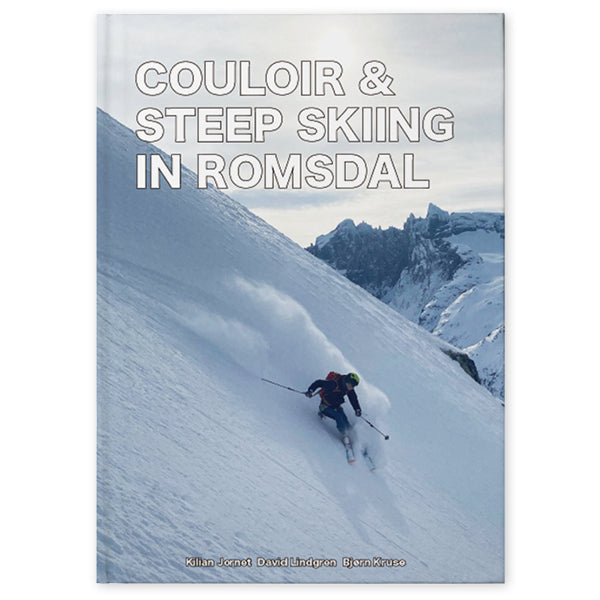The book cover features a dynamic image of a skier gliding down a smooth, snow-covered mountainside, leaving a trail of snow in his wake as he moves from the left to the right. In the background on the right side, another rugged, rocky mountain peaks through, partially covered in snow, under a cloudy sky. At the top of the cover, bold white text with a red border reads "Couloir and Steep Skiing in Romsdal." At the bottom, the authors' names, Killian Jornet, David Lindgren, and Bjorn Kruse, are listed in smaller white text. The image captures the thrilling essence of skiing in a dramatic alpine setting.